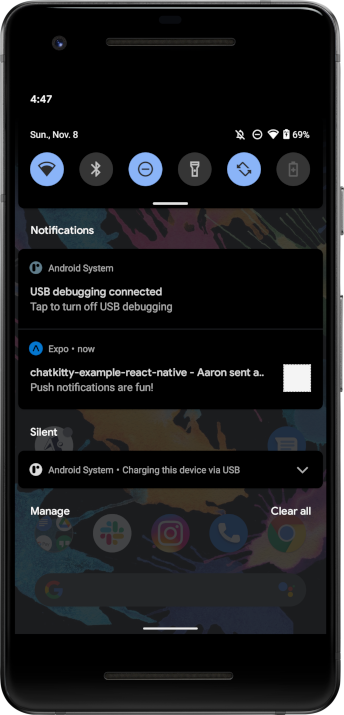The image depicts a sleek black cell phone with several distinct features. The right side of the device showcases its volume up and down buttons alongside the power button, all emerging subtly from a slight indentation. The top and bottom portions of the phone exhibit a glossy, reflective quality. At the top center, there is a small circular camera and a horizontal line that likely functions as a speaker.

In the upper left-hand corner of the phone's display, the time reads 4:47, and below it, the date is Sunday, November 8th. Various status icons are visible, including Do Not Disturb, Wi-Fi, and Battery Life at 69%. The user interface displays additional icons such as Bluetooth, flashlight, auto-rotate, and battery saver. The wallpaper features a vibrant paint splatter design in red, yellow, blue, and black.

Furthermore, a notifications panel is partially visible. Notifications include system alerts such as "USB debugging connected" with an option to turn it off, "Expo Now," "Chat Kitty," "Example React Native errands that day," "Push notifications are fun," "Silent," "Android system charging this device via USB," and options to manage or clear all notifications.